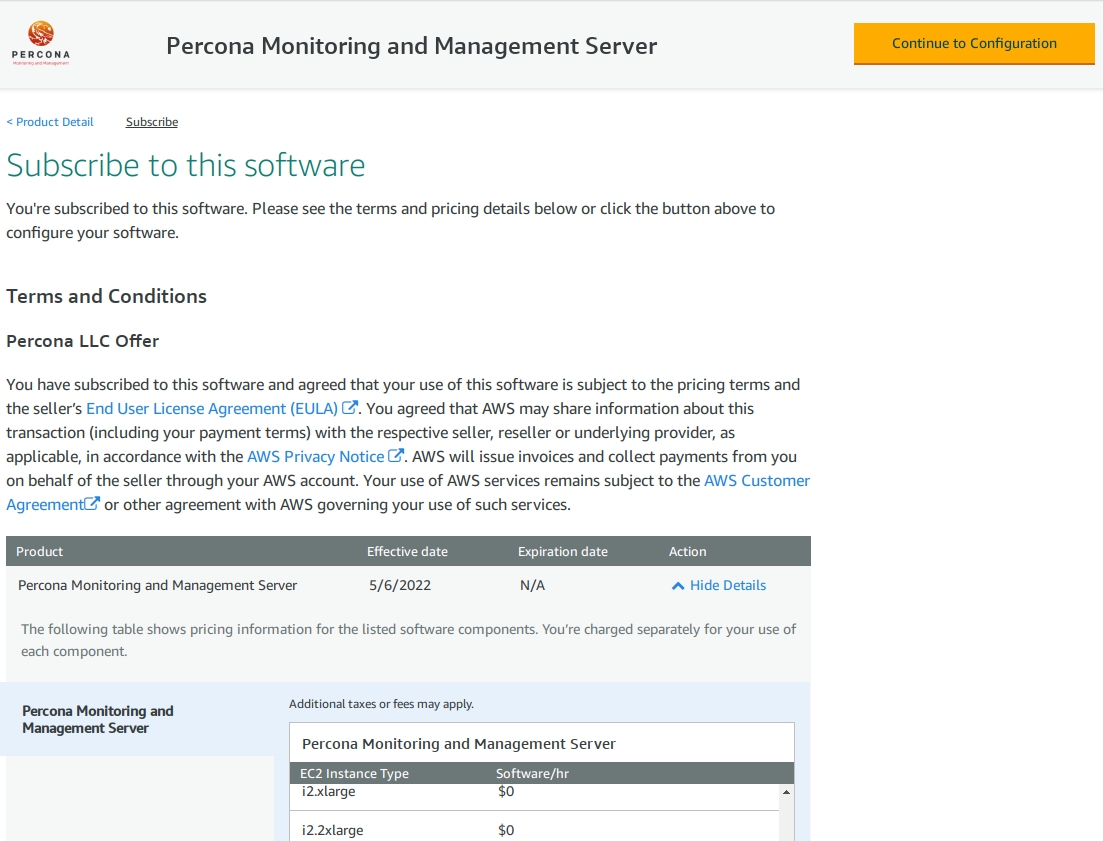The image depicts a screen from a Percona Monitoring and Management Server interface. Prominently featured is the Percona icon, a round circle with a yellow-orange gradient resembling a globe. At the top, an orange button is labeled "Continue to Configuration." Below this button, bold text reads "Product Detail."

Next, there is a black header titled "Subscribe" with a blue underline. In teal text, the interface displays "Subscribe to this software." Further down, a notification in standard text states, "You are subscribed to this software. Please see terms and pricing details below and click the button to configure your software."

Additional text on the screen presents terms and conditions, including a mention of "Percona LLC Offer." It confirms, "You’ve subscribed to this software and agreed that your use of this software is subject to the pricing terms and the seller's end user license agreement."

Links in blue text are provided for the "Privacy Notice" and "Customer Agreement," allowing users to view these documents.

Another section provides specifics in a grid format:
- **Product**: Percona Monitoring and Management Server
- **Effective Date**: 5-6-2022
- **Expiration Date**: N/A
- **Action**: A blue hyperlink labeled "Hide Details"

Finally, a note confirms the purchase of the software and describes its type, emphasizing its management and monitoring capabilities.